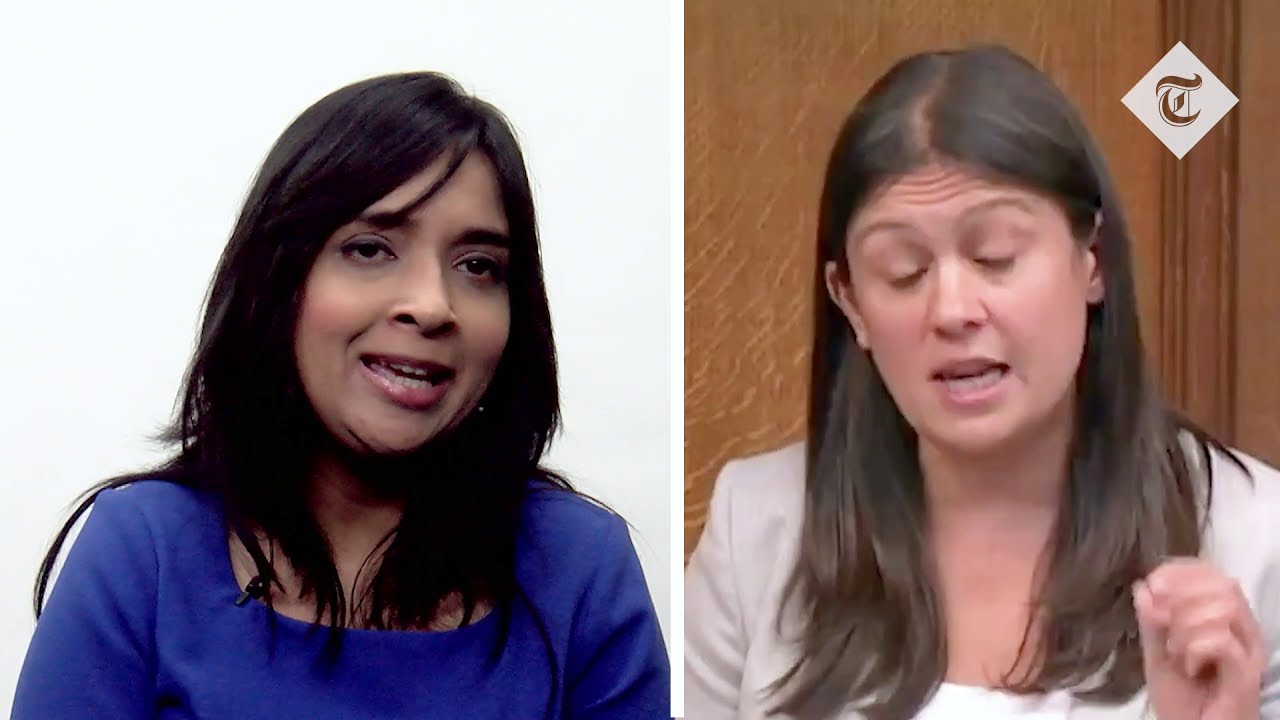This image features two side-by-side photographs, each depicting a woman as if they are engaging in a dialogue or critique, reminiscent of a webcam interaction. On the left is a woman with medium brown skin and long, dark hair, possibly of Middle Eastern descent. She is dressed in dark, possibly formal attire that includes a black or dark blue top. The background is stark white, and she appears to be looking slightly to the right of the viewer, her mouth slightly open as if caught mid-sentence.

On the right is a white woman with long brown hair, dressed in a gray and white blouse. She has her eyes closed and her hand raised, as though emphasizing a point. Behind her is a wooden wall with some etching, evoking an environment like that of a courtroom. In the upper right corner of her image is a distinctive emblem—a white 'T' in a blue diamond, resembling the New York Times logo. Both women, though in separate images, appear to be captured in moments of expressive communication.